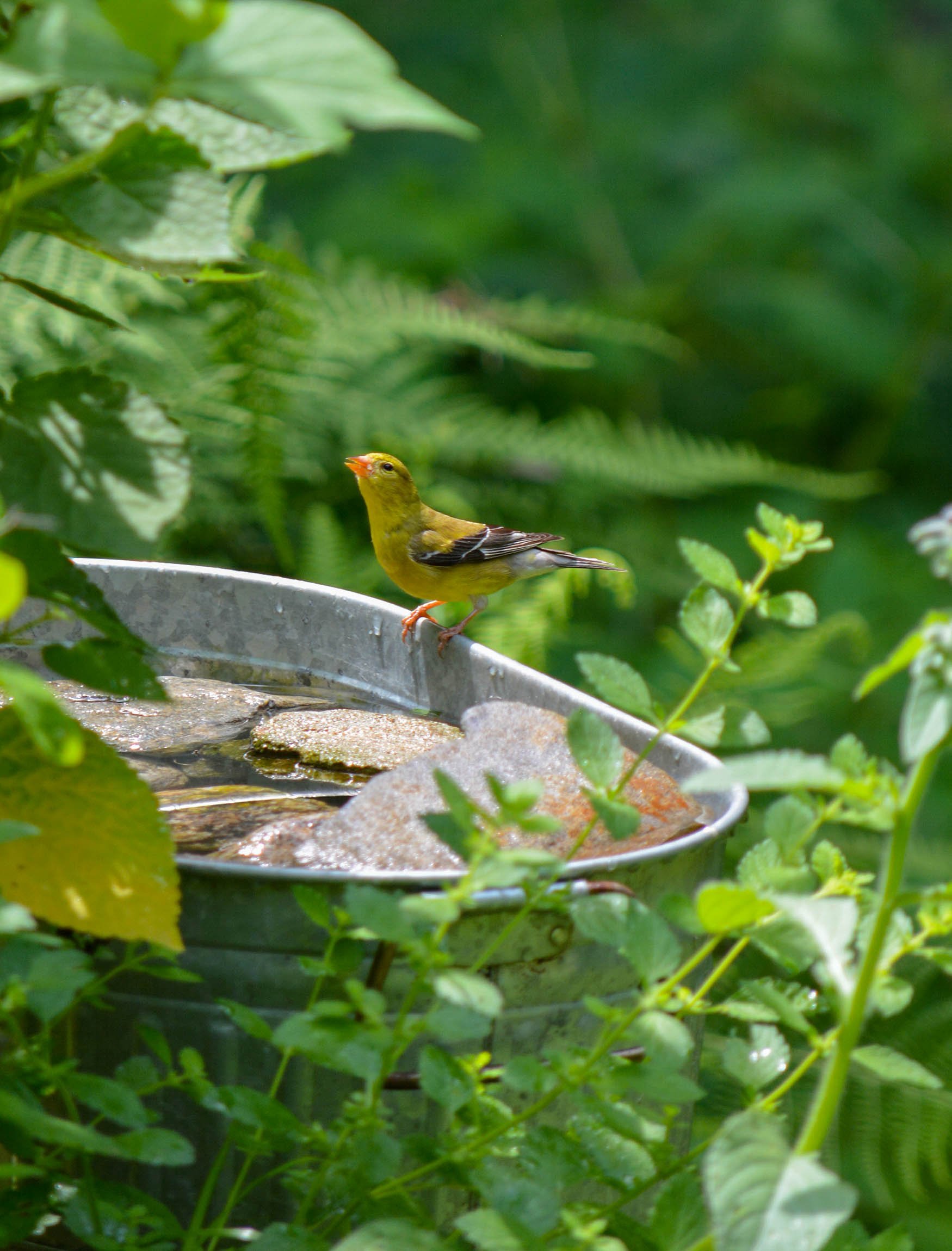In this vibrant, color photograph, a close-up captures a lively scene centered around a small yellow bird perched on the edge of a silver, galvanized iron bucket, serving as a bird feeder. The birdbath is filled with flat stones and a considerable amount of water. The bird, displaying a vivid yellow and brown body, has a distinguishing sharp, short, bright orange beak and captivating black eyes accentuated by a small white spot on its forehead. Its wings are a striking mix of black and white feathers, and its tail mirrors this pattern with predominantly white feathers. The bird’s feet are an orange hue, firmly gripping the bucket's edge. In the background, the lush green foliage, a mix of ferns and various leafy plants, provides a beautiful, blurred backdrop under the sunlight, enhancing the serene, natural setting. The intricate details of the bird and its surroundings are captured, showcasing a harmonious blend of nature's colors and textures.